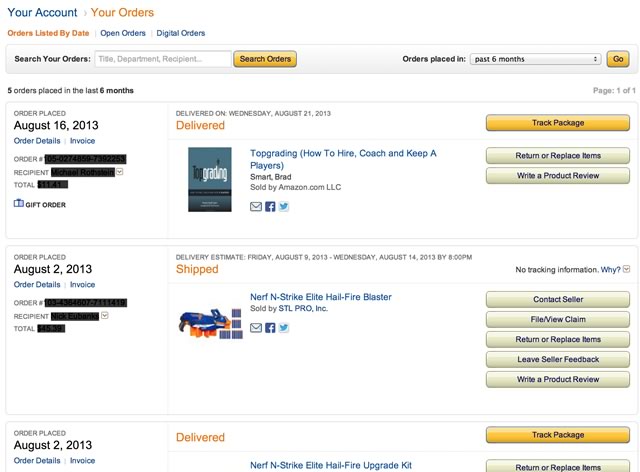The page features a user account summary in the upper left corner, adjacent to the order section on the right. The order section is itemized by categories including "orders listed by dates," "order," "open orders," and "digital orders." Directly below these categories, you'll find a search functionality comprising a search field and a yellow "Search Orders" button. 

To the right on this row, a dropdown menu allows users to filter "Orders placed in" specific time frames, such as the past six months, followed by a yellow "Go" button. Under this, the section lists orders placed in the last six months, detailed by date and status. 

The order history displays the most recent entries:
- August 16th, 2013: Order delivered.
- August 2nd, 2013: Order shipped.
- August 2nd, 2013: Order delivered.